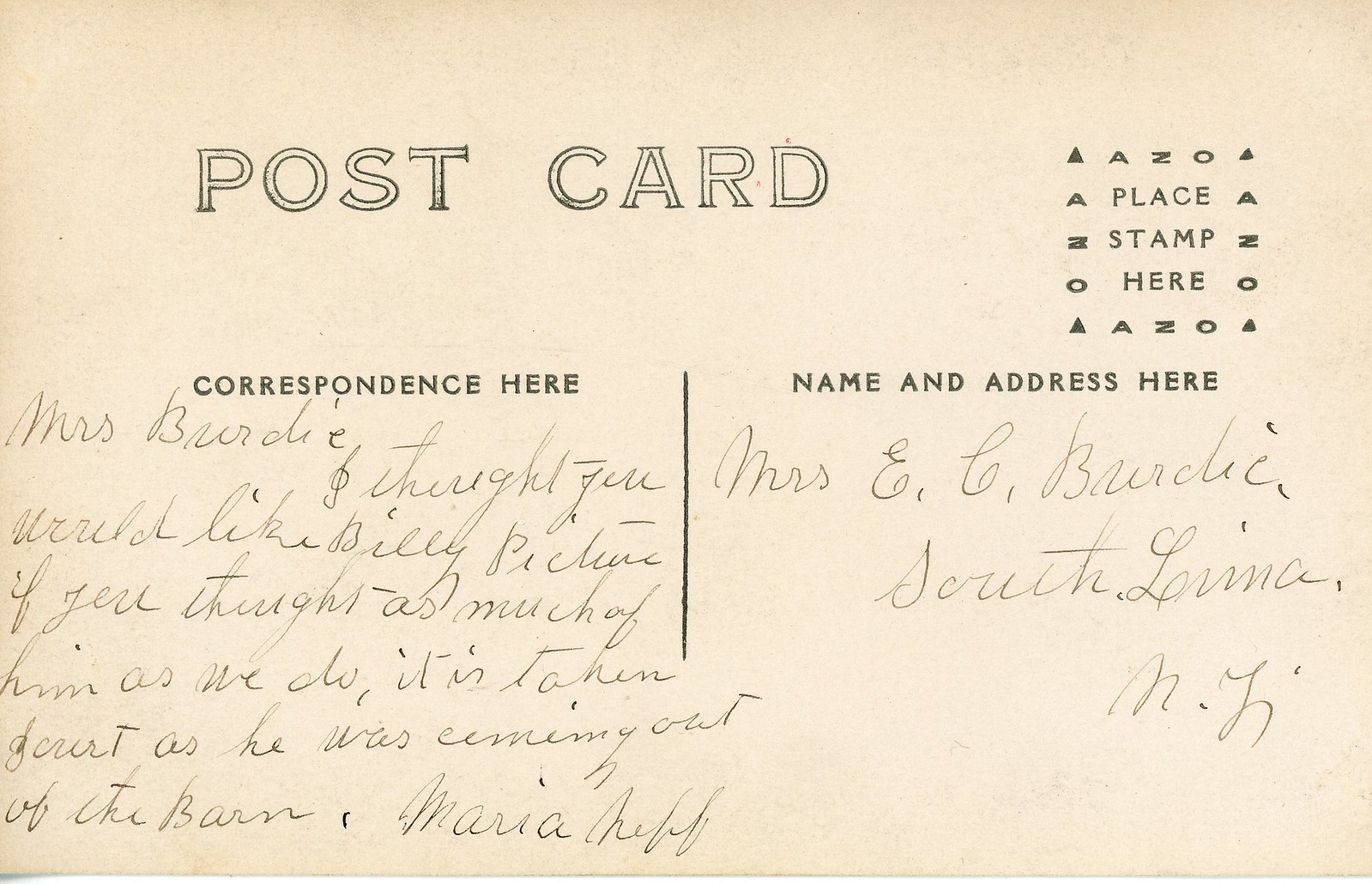The image depicts the back of an old-fashioned postcard with a thick white border. At the top, the word "POSTCARD" is written in bold, uppercase two-line black characters, set against a very pale pink background. In the top right corner, there is a designated square for placing a stamp, which reads "Place Stamp Here." 

Below this, the postcard is divided into two sections. On the left, under the heading "Correspondence Here" in blue text, a handwritten message in cursive reads, "Mrs. Brody, thank you. Thought you would like Billy's picture if you thought as much of him as we do. It is taken just as he was coming out of the barn." The letter is signed by Maria Huff.

On the right side, under the heading "Name and Address Here" in blue text, the recipient's name and address are written: "Mrs. E.G. Brody, South Lima, New Jersey."